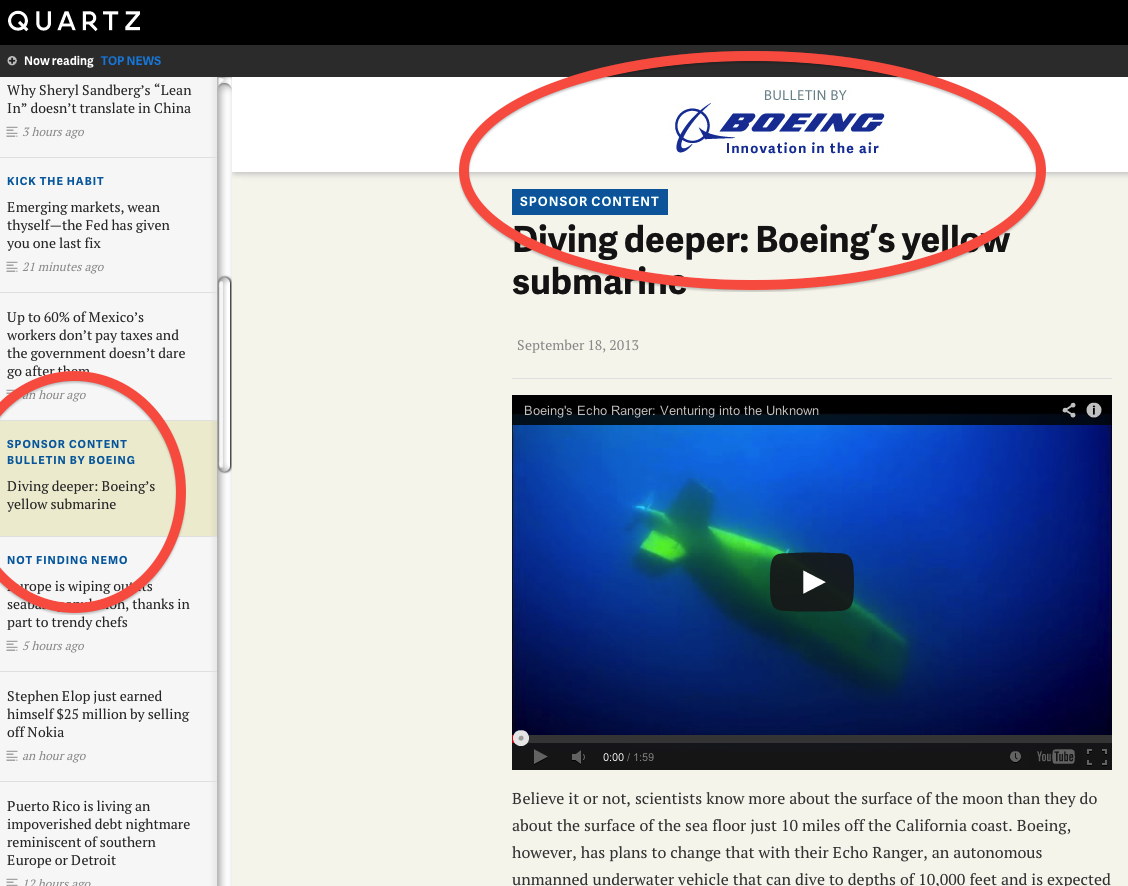This image is a screenshot from a webpage, with specific sections highlighted by red oval borders. Across the top from the upper left to the upper right is a black stripe that reads "Quartz." Below it, text reads "Now Reading," followed by a blue-highlighted "Top News."

On the left side of the image, several headlines are listed in a column. They include:
- "Why Sheryl Sandberg's 'Lean In' Doesn't Translate in China"
- "Kick the Habit: Emerging Markets, Wean Thyself, The Fed Has Given You One Last Fix"
- "Up to 60% of Mexico's Workers Don't Pay Taxes and the Government Doesn’t Care to Go After Them"
- "Sponsor Content: Bulletin by Boeing – Diving Deeper: Boeing's Yellow Submarine"
- "Not Finding Nemo: Europe is Wiping Out Something"
- "Stephen Elop Just Earned Himself $25 Million"
- "Puerto Rico is Living in an Impoverished Debt Nightmare Reminiscent of Southern Europe or Detroit"

Additionally, the displayed content indicates "Top of 12 Hours," suggesting recent or significant news.

Adjacent to this column, on the right, there is a vertical menu bar, indicating the page is scrollable. The sponsor content "Bulletin by Boeing" is highlighted, noting "Innovation in the Air" and "Diving Deeper: Boeing's Yellow Submarine." The prominent mention of Boeing is intriguing, particularly in the context of the company's well-known challenges.